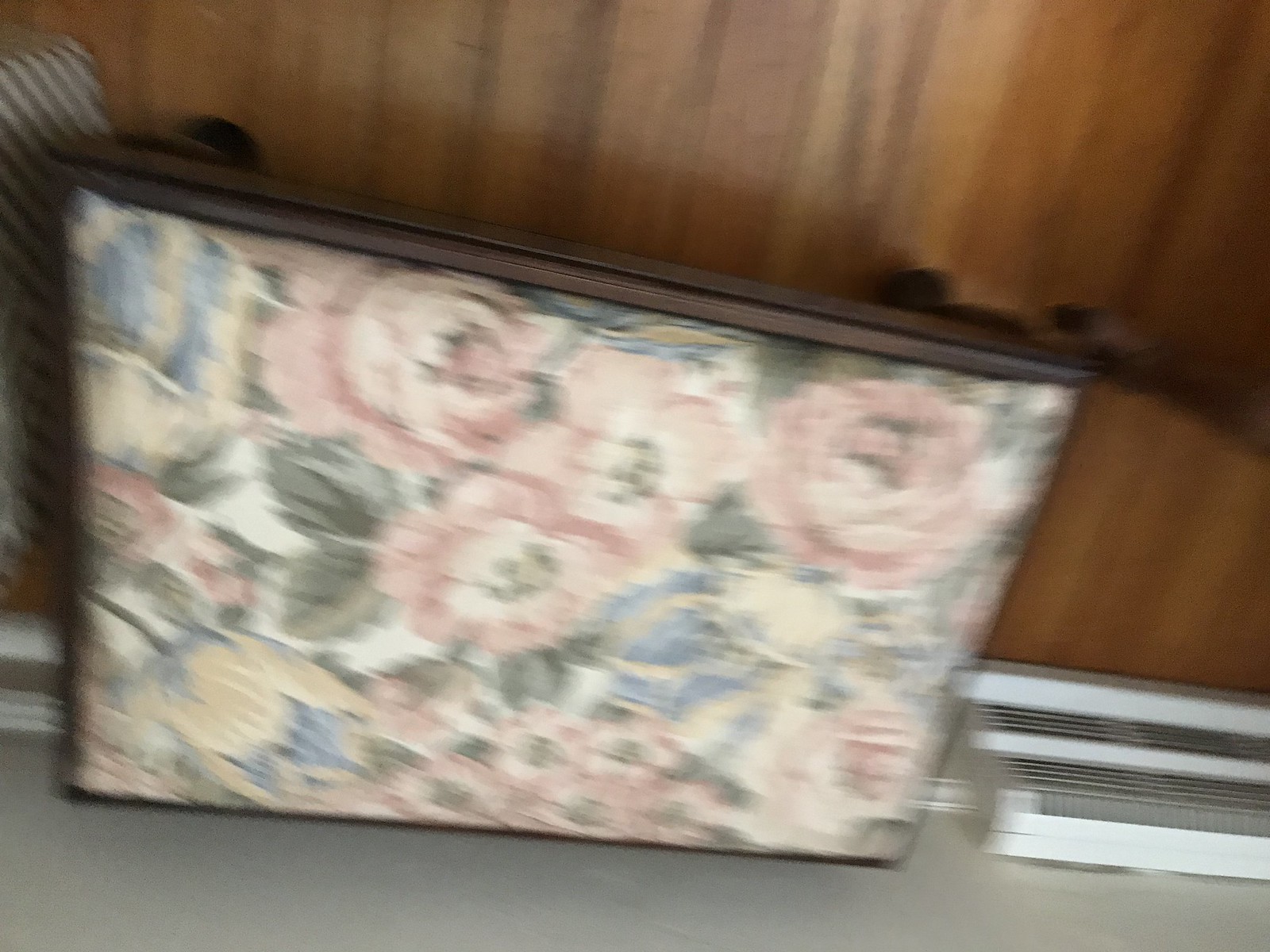This is an exceptionally blurry image that appears to feature a floral-upholstered hassock seen from an unusual, likely sideways perspective. The blurred object rests on a hardwood floor displaying dark and light brown tones. The wall, appearing in the lower part of the image due to the sideways orientation, is gray with a visible air conditioning vent to the left.

The primary focus is a hassock with dark brown wooden legs and an upholstery adorned with a vintage floral design, including pink cabbage roses accompanied by green leaves. The upholstery also features blue and tan flowers, although the exact type of the blue flowers is hard to discern due to the blurriness. There are suggestions that the top of the hassock may have a stained wood aspect, which adds to its aged, classic appeal. Overall, the detailed floral pattern and the vintage feel of the object make for a unique yet indiscernible focal point in this poorly captured image.